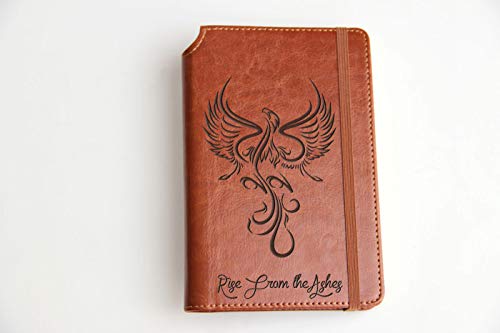The image features a beautifully crafted leather notebook set against a solid white background. The notebook, resting on what appears to be a table, boasts a rich ember red color with a subtle reddish-brown hue. Its design includes a unique half-circle notch on the top left corner, adding to its distinctive appearance. The right corners are rounded, enhancing the sleek, well-crafted look. A leather strap wraps around the book, securing it together, and white thread is intricately stitched around the binding, suggesting high craftsmanship and possibly an expensive piece.

The notebook's cover is adorned with a detailed black carving of a phoenix, with clearly visible wings, head, and an intricate, line-based body design. Beneath the phoenix, the phrase "Rise from the Ashes" is elegantly inscribed in black cursive, with each initial letter—R, F, and A—capitalized. The overall image is simplistic, emphasizing the notebook as the focal point, highlighting its creative and artistic qualities.